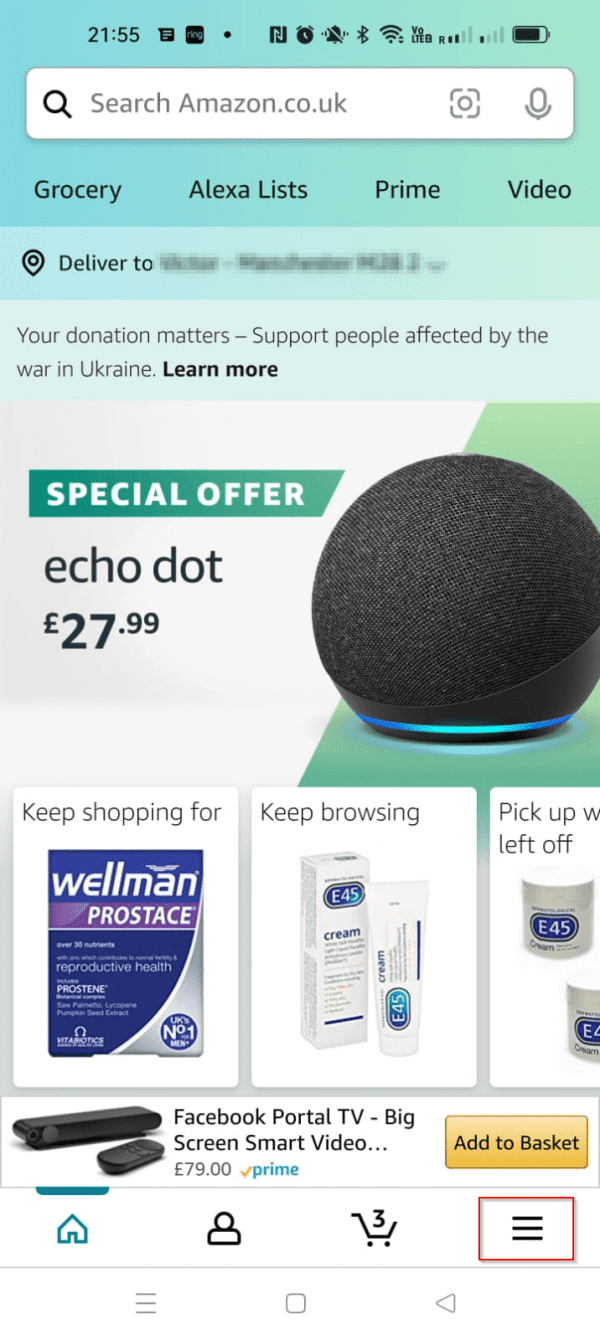This image captures a screenshot from a cell phone displaying the Amazon.co.uk search page. The background of the page is predominantly teal with some white accents. The user appears to be viewing a special offer for the Echo Dot, priced at £27.99. The Echo Dot is visually represented as a small, black, spherical device.

Prominently displayed on the page is a message encouraging donations to support people affected by the war in Ukraine, accompanied by a "Learn More" link. Below this, the page prompts the user to "Keep shopping for" Wellman Prostase, presumably a previously viewed item. Further down, there is a suggestion to "Keep browsing" for E45 cream, indicating another recent search or shopping interest.

At the bottom of the screen, a suggestion to "Pick up where you left off" appears, also referencing the E45 cream. Additionally, there is a mention of the "Facebook Portal TV - Big Screen Smart Video" which seems to be another product previously considered by the user. The "Add to Basket" button is visible, highlighted in a yellowish-orange box.